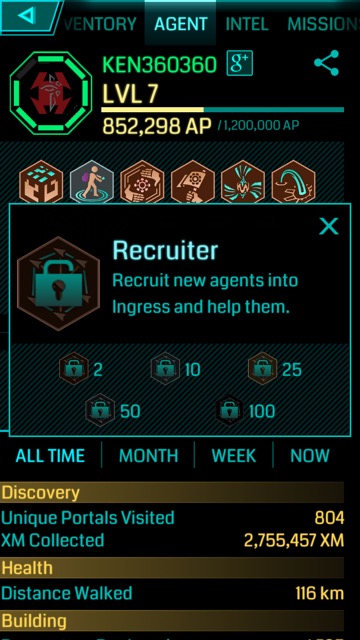The image appears to be a screenshot from a mobile game interface, showing the "Agent" section. At the top, there is a navigation bar with clickable options: Inventory, Agent (currently selected), Intel, and Mission, along with a back button. Below this, the player's username, Ken360360, is displayed in green, accompanied by a Google Plus logo to the right. The player, currently at level 7, has an AP (Action Points) bar indicating they are nearly halfway to the next level. Centrally located is a box labeled "Recruiter," which reads "Recruit new agents into Ingress and help them," yet this ability is locked, as indicated by a padlock icon on the left. At the bottom of the screen, there are tabs labeled All Time, Month, Week, and Now, providing detailed stats such as Health and Distance Walked. The screen's design features well-organized elements with various colors, including light blue, black, red, peach, and yellow, enhancing the clarity and aesthetics of the mobile game interface.